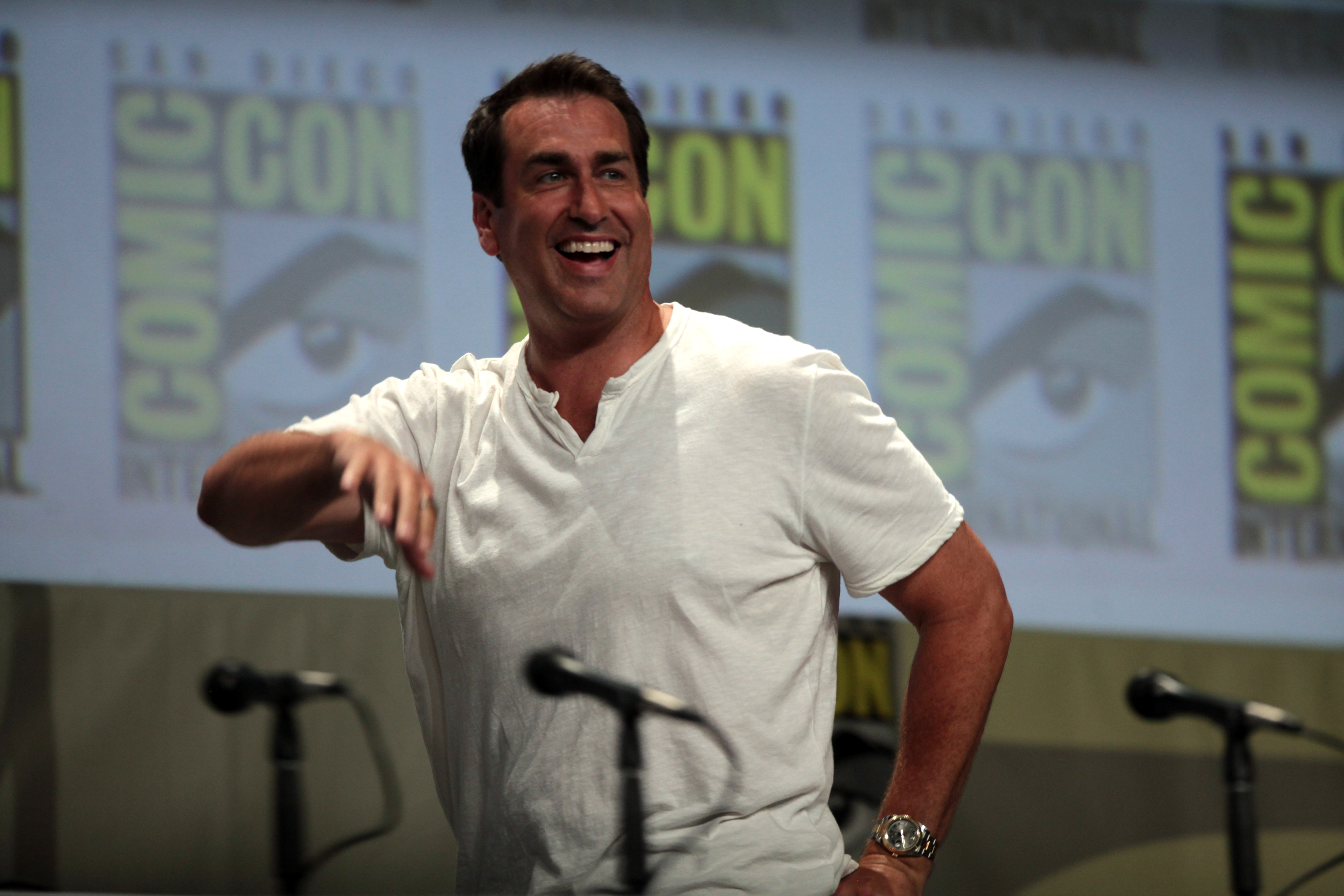In the image, we see Rob Riggle, also known as Robert Allen Riggle Jr., a well-known actor and stand-up comedian, standing at what appears to be a San Diego Comic-Con event. Rob has short dark hair parted to the side, which is slightly receding. He is wearing a light-colored, short-sleeved v-neck t-shirt and a silver watch. With a broad smile, his mouth is open, revealing his top row of teeth. His right arm is bent and raised, possibly gesturing to or waving at the audience, while his left hand rests on his waist. In front of him are a few microphones, blurry and out of focus, indicating he is either walking onto or off the stage. The background features a banner repeating the text “Comic-Con” in green print along with an image of an eye and eyebrow, setting the scene unmistakably at the famed convention.